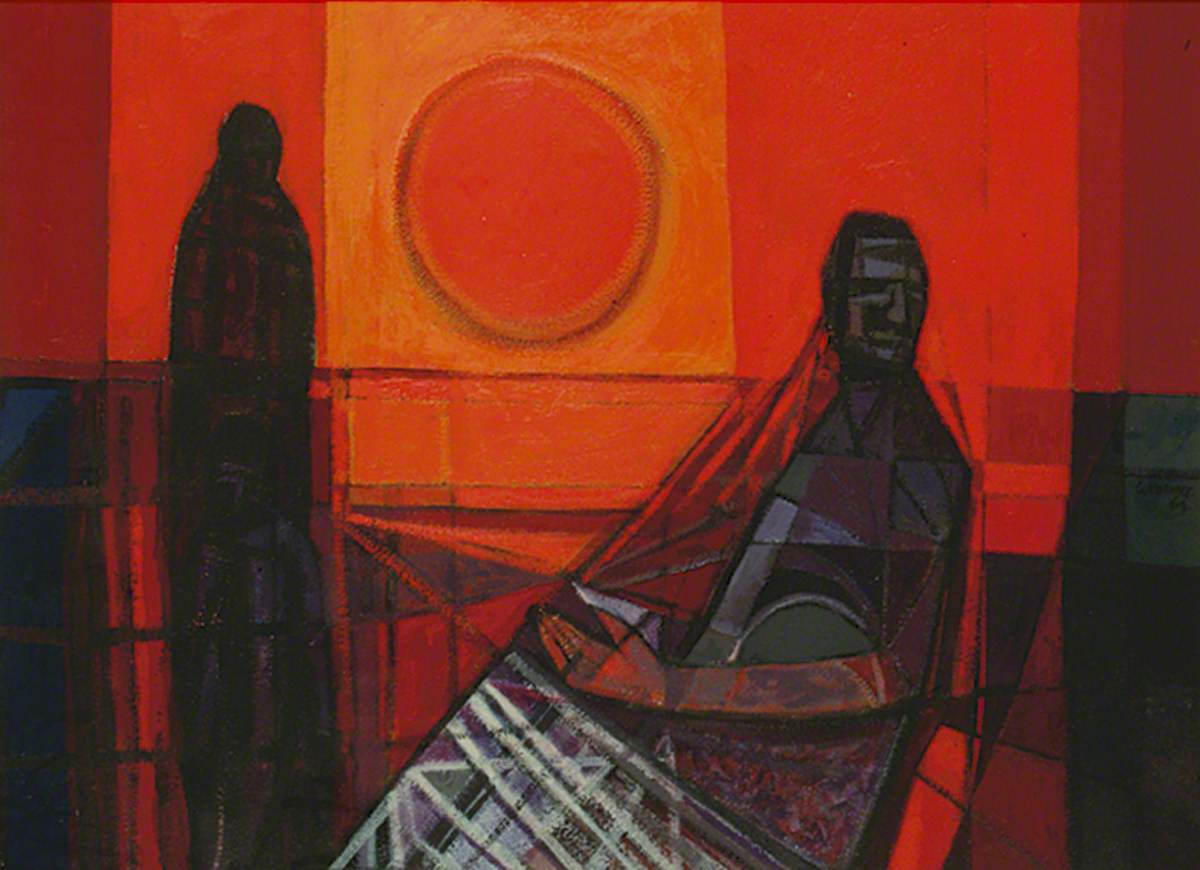This abstract painting features a vivid scene dominated by bold geometric shapes and a warm color palette. The background transitions from deep red to vibrant orange, framing a large circular sun in the center, outlined in dark gray. The scene appears to depict two figures against this sunset-lit backdrop. On the right, a person is rendered in an impressionistic style with black facial features and a body composed of angular triangles and straight lines, with an arm crossing their torso. This figure gazes back over their left shoulder, possibly holding an abstract object like a net. To the left, a tall, shadowy figure with an indistinct profile stands, contributing to the painting's mysterious and dynamic composition. The overall effect is an evocative blend of red, orange, black, and hints of purple, creating a visually striking and thought-provoking piece that captures the essence of human interaction within a fantastical landscape.